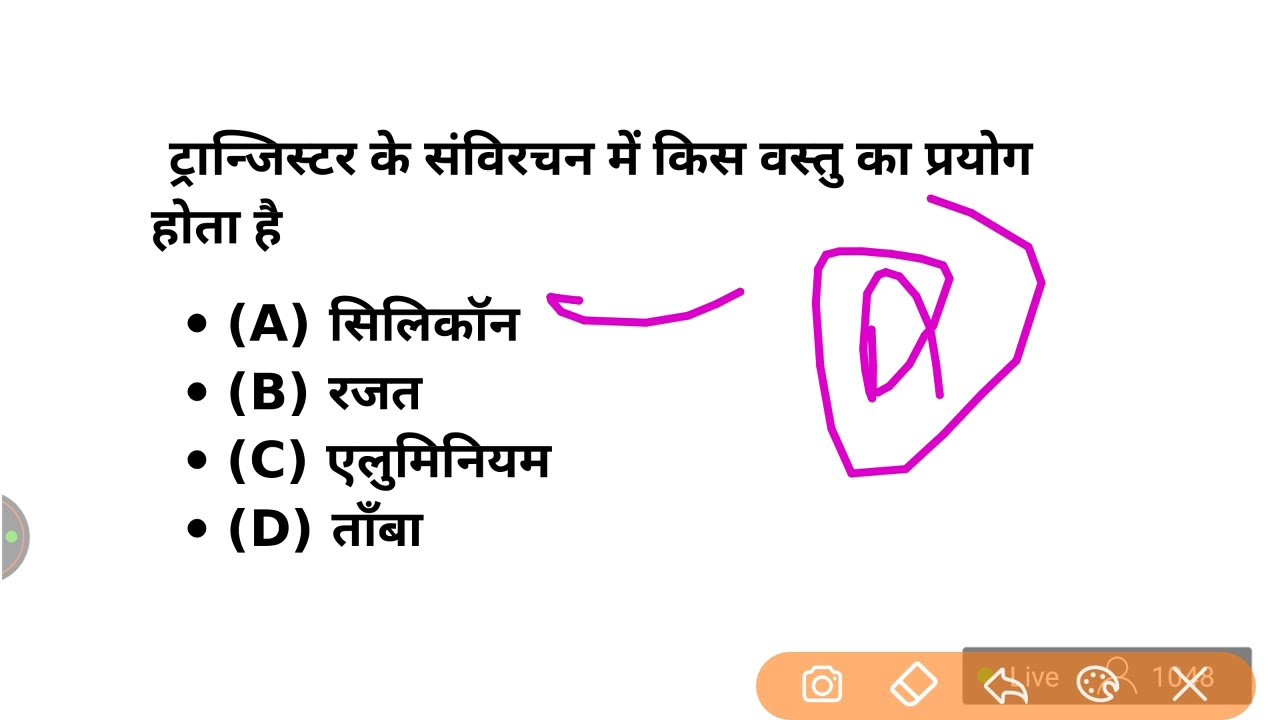The image is a landscape-oriented screenshot, likely from a website or a mobile device. The background alternates between black and white and features a prominent heading in Arabic script at the top. Below the heading are four bulleted choices labeled A, B, C, and D, each followed by more Arabic text. Highlighting one of the bulleted options, specifically line A, is a purple circle resembling a bullseye with an arrow pointing towards it, suggesting it might be the correct answer. In the lower right corner, an orange rectangle contains social media icons, including an Instagram camera, a square, an arrow, a paint palette, and an X. The screen also includes a navigational panel at the bottom, consisting of five symbols, indicating different functionalities for navigating the page.